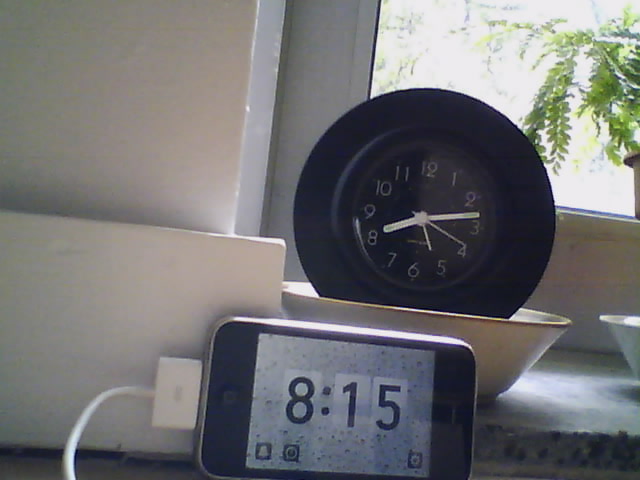The image captures a detailed scene featuring two timepieces on what appears to be a bathroom countertop. The first timepiece is a small, round, black analog clock with white numbers and hands, displaying approximately 8:13. This clock is nestled inside a white ceramic dish with a gold rim. In front of it lies an older model iPhone, possibly an iPhone 6, laid on its side and plugged in; the digital clock on the phone reads 8:15. To the right of these items, there is another small bowl partially visible. The background includes a tan wall with white trim and a window that allows sunlight to illuminate the scene, revealing green leaves and branches from a tree outside, indicating a sunny day.